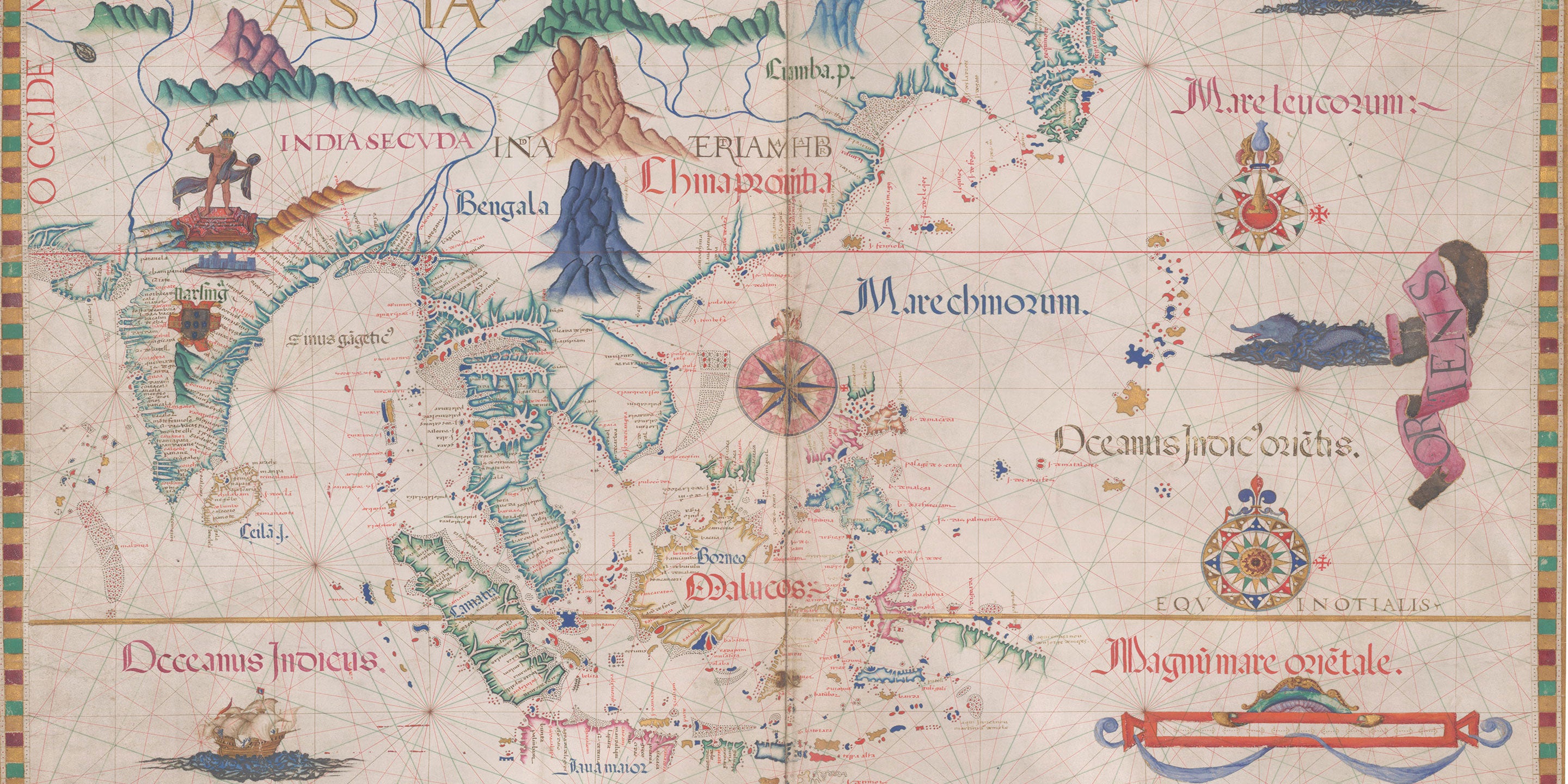The image presents an artistically rendered, historically styled map, possibly from the 17th century, adorned with a variety of vibrant colors and intricate illustrations. The map features landmasses and names such as Marci, Co-Rim, Marley, Co-Lim, Dorcas, Indicus, India, and Secunda, suggesting a blend of fantasy and foreign influences. The language appears ambiguous, with possible traces of Latin or Spanish, and includes terms like "Oceanus Indicus" in red. Key elements include detailed depictions of mountain ranges in vivid hues—purple, brown, and green—as well as a multitude of colorful banners, islands, and a ship situated at the bottom left. Central to the composition is a compass, while the top left mentions "Oxidide," perhaps indicative of the Occident. Additionally, illustrations such as a horseman and a figure standing on a temple enrich the visual narrative, alongside terrains marked as Bengala with distinctive blue and brown mountains. The water bodies diverge from the conventional blue, enhancing the map's unique artistic character.